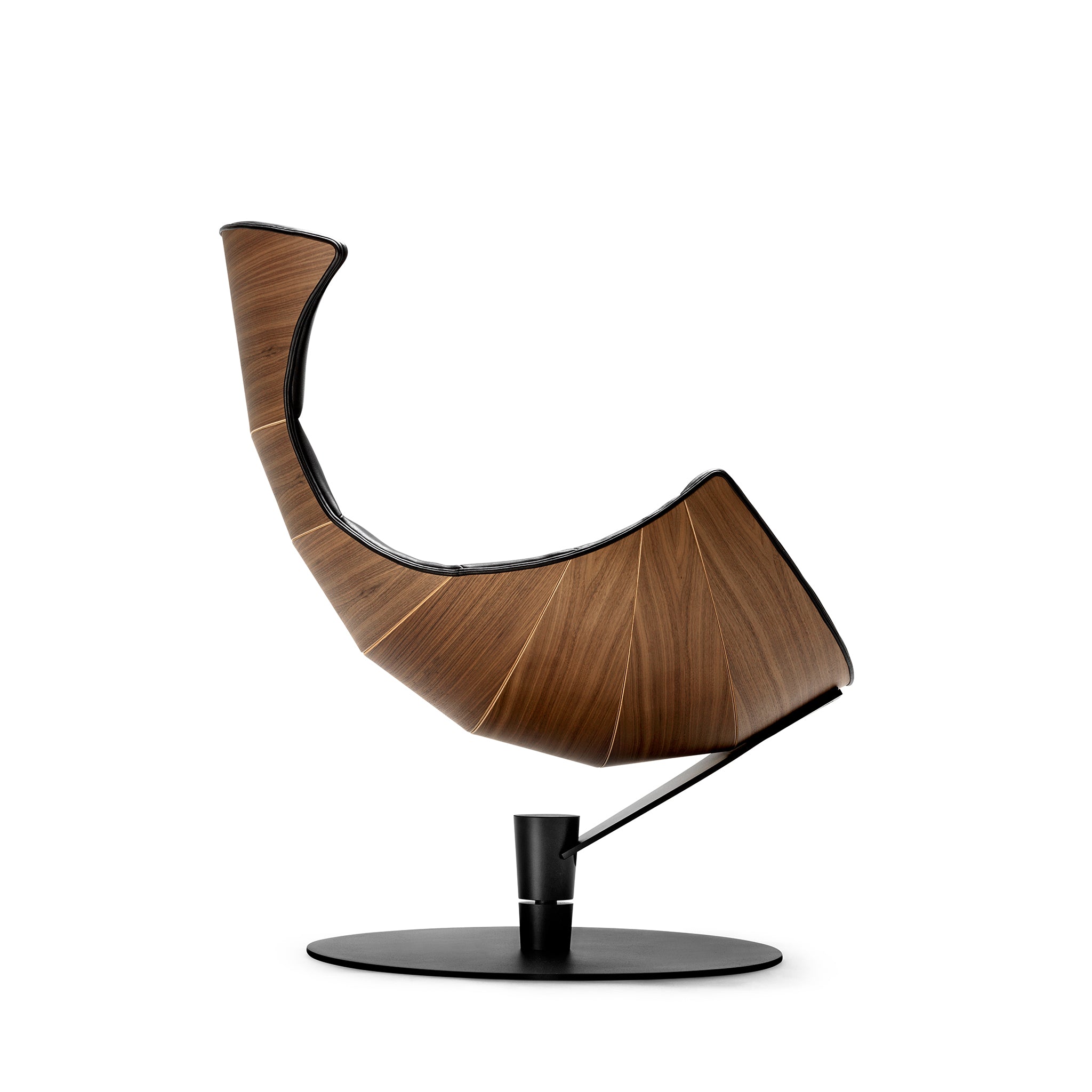This vertical image showcases a uniquely modern chair designed to pivot, positioned on a sleek black metal base. The base is a glossy, round plate with a central protrusion that supports the chair through a connecting metal arm, allowing for 360-degree rotation. The chair itself is crafted from slatted, laminated wood, forming a deep brown, acorn or horn-shaped shell that narrows towards the top. Its basket-like, curved design suggests it may be challenging to sit in and get out of, as the primary support is located at the very front, creating an impression of instability. The innovative, sculptural appearance of this chair makes it a striking and unconventional piece of furniture.